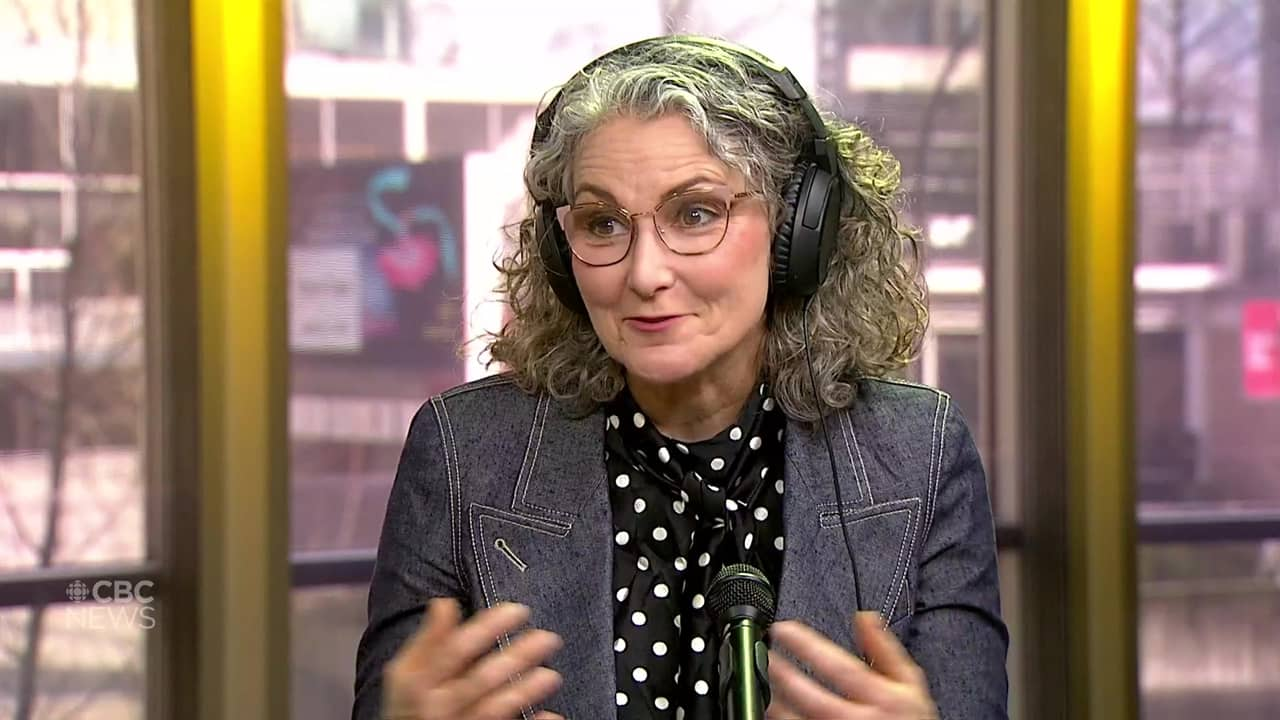The image features an older woman, possibly in her 60s, seated and speaking into a black microphone positioned in front of her, suggesting she might be part of a podcast or interview show. She has voluminous, wavy gray hair possibly styled with product, and she wears wire-framed glasses that are slightly pointed where the arms meet the lenses. She is dressed in a dark bluish-gray denim blazer, underneath which she sports a shiny black blouse adorned with white polka dots and a bow tie. Her ensemble is complemented by light makeup, including pink lipstick and a touch of blush on her cheeks. The woman also has black, over-ear wireless headphones on, and her expression is intent and engaged, as if explaining something. In the backdrop, large metal-framed glass windows reveal a cityscape with buildings, trees, and some signage. Notably, the lower left corner of the image displays the hashtag #CBCNews, denoting that the scene is likely associated with the Canadian Broadcasting Corporation (CBC).